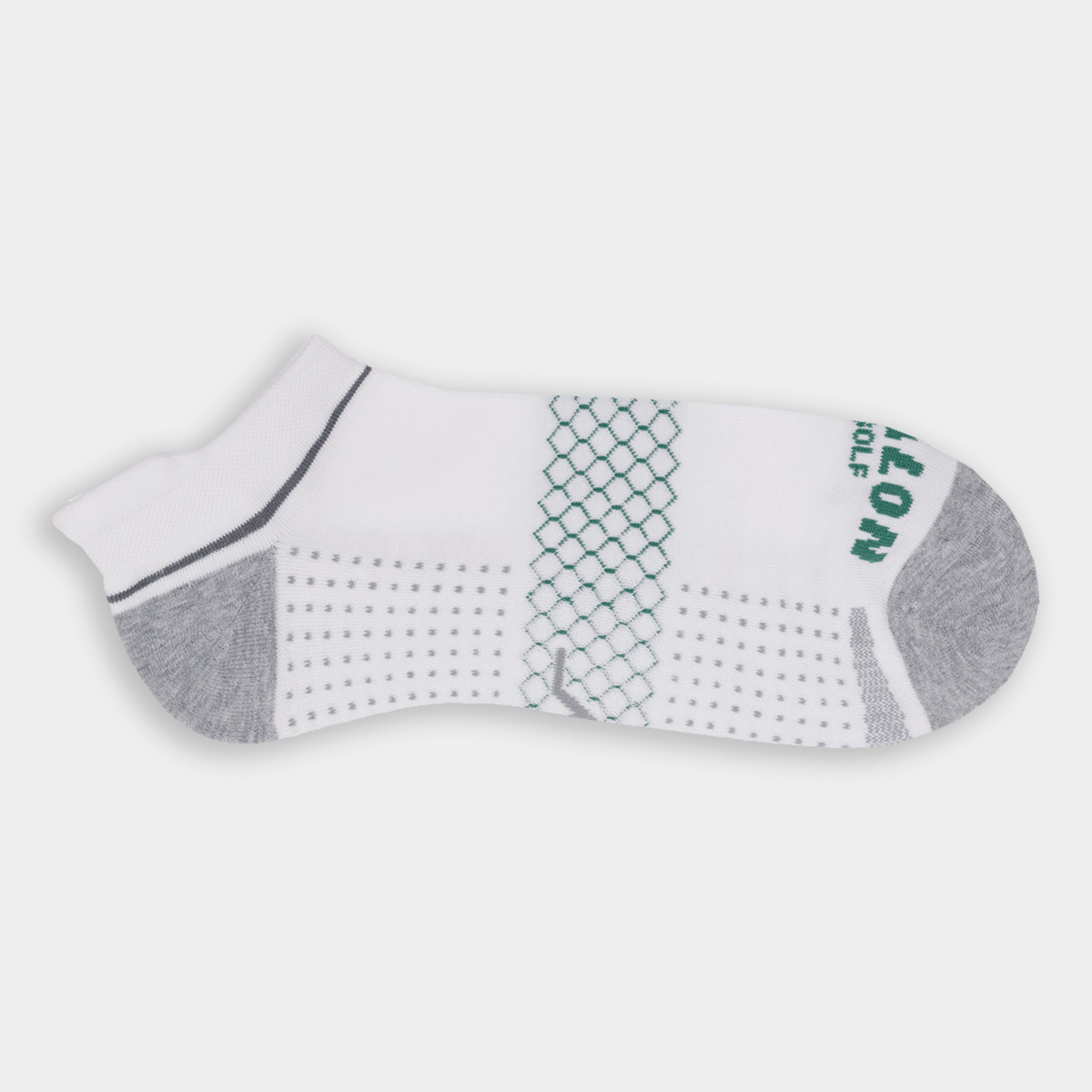This image features a single ankle sock positioned centrally against a solid white background. The sock itself is primarily white with a very low cuff. A black line encircles the sock about an inch below the cuff. The sock also features a light heather gray heel and toe, with additional gray accents at the front tip and a thick gray line along the bottom. Along the sole, you'll find gray dots, which add to the detailed design. Running down the center of the sock is a stripe composed of green diamond shapes with white interiors, creating a fish scale or netting appearance. Near the tip, just beside the gray area, there's green text—partially viewable due to the sock's positioning—that reads "L-O-N" above "O-L-F," likely referring to the word "golf." The image is brightly lit and the details are clearly visible, emphasizing the distinct colors and patterns of the sock.